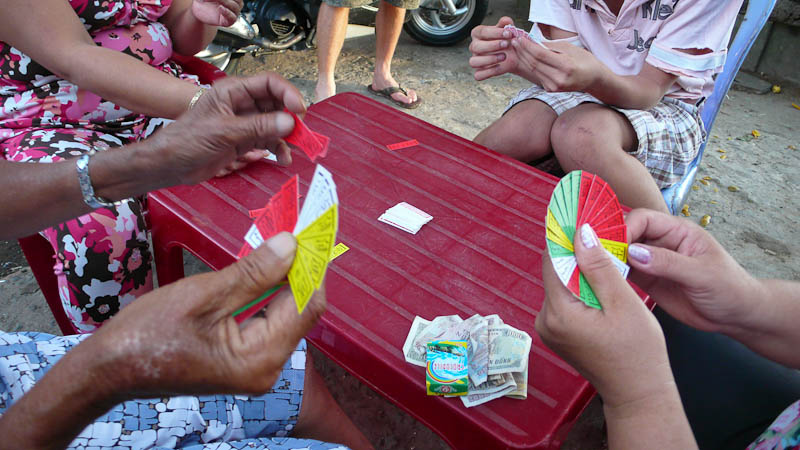In this landscape-mode photograph, four people are engaged in a game that appears to involve money. The scene is centered around a small plastic table. 

In the upper left-hand corner, a woman with tan skin is wearing a distinctive pink and brown dress. Moving along the lower-left center to the lower-right center, there's another individual with darker hands adorned with a bracelet on the left wrist. This person has white spots on their right hand and is dressed in a blue and white patterned outfit. 

In the bottom right-hand corner, a person with tan hands and pink nail polish is visible. The upper right-hand section reveals an individual wearing a shirt with tears in it, paired with brown and light blue shorts. It is unclear whether the tears are a fashion statement or from wear and tear. In the upper center, another person, identifiable by their light skin, is dressed in brown flip-flops and shorts.

The table itself, particularly the bottom right-hand corner, is cluttered with a substantial amount of green bills. Amidst the money sits a green and yellow box, likely used for storing game-related items. Scattered across the table, red, white, and yellow tags that resemble tickets can be seen, indicating these might be crucial to the mysterious card game being played. Despite the vivid details, the nature and rules of the game remain unclear.